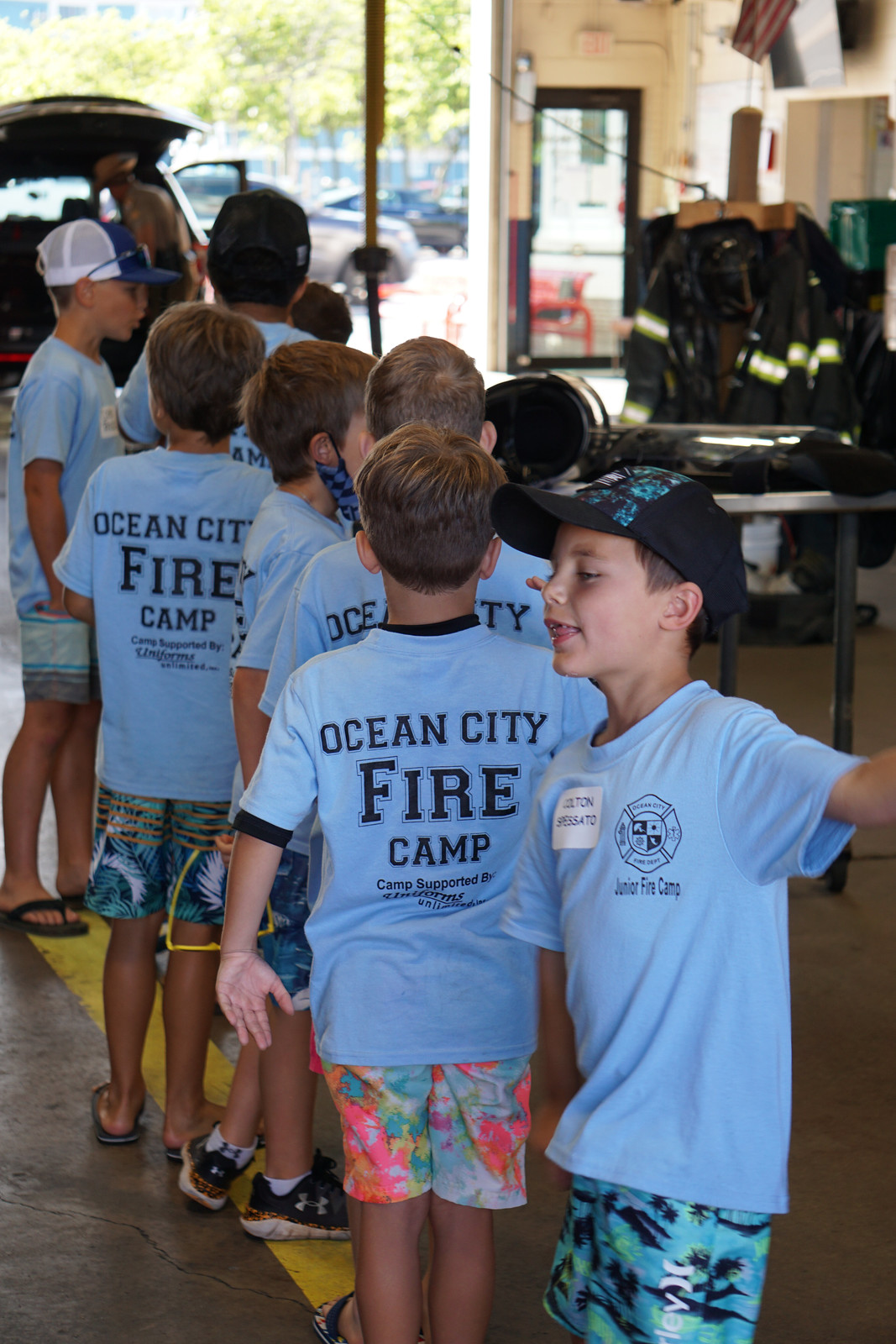In this vibrant photograph, a group of approximately nine to ten young boys, estimated to be between the ages of 7 to 10, are standing in front of a firehouse, their backs turned to the camera. Each boy is donned in a matching light blue t-shirt emblazoned with the words "Ocean City Fire Camp" in black letters, and an indistinguishable logo over the left breast. They are dressed in an eclectic mix of tropical printed Bermuda shorts and colorful shorts ranging from blue and black to red, pink, orange, and yellow. Footwear varies from sneakers to flip-flops. Two boys sport baseball caps, and one holds a pair of yellow sunglasses.

The setting suggests a lively waiting line, possibly for a fire camp activity, given the firehouse environment, with visible fire uniforms, equipment, hoses, and extension cords in the background. The scene is bright and sunny, underscored by the sight of an open parking lot and the open bays of the firehouse. Additionally, there is a vehicle with open doors and luggage, hinting that the boys might be preparing for an outing. This image captures the spirited anticipation and camaraderie among the young campers.